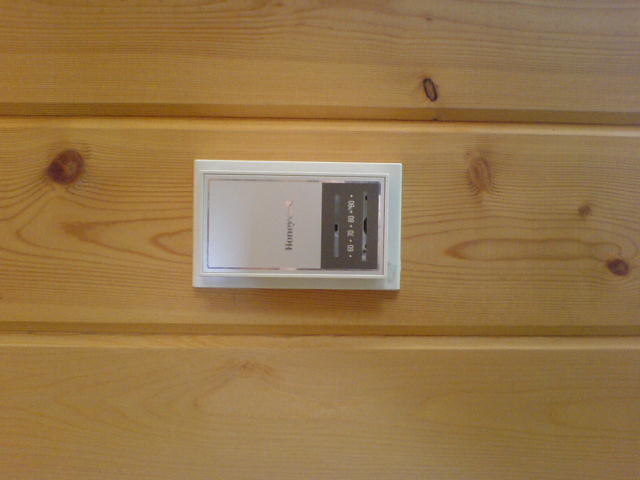The image features a Honeywell thermostat mounted on a wall made of light knotty pine planks, positioned horizontally due to the sideways orientation of the photograph. The thermostat is centrally located on the middle plank among the three visible planks. It is white and rectangular in shape.

The thermostat design includes an outer rectangular frame and an inner rectangle where the brand name "Honeywell" is prominently displayed in silver in the center. On what is the right-hand side of the sideways image, the thermostat displays temperature settings marked as 60, 70, 80, and 90 degrees. A small slider is visible for adjusting the temperature. Additionally, there are little slits located above and below the temperature numbers, but their specific function is unclear, though they might be related to the thermostat's internal mechanisms.